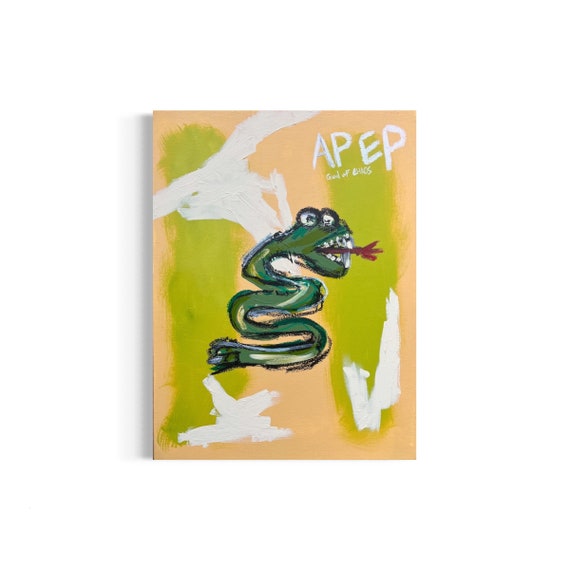This small, vertical rectangular painting features a cartoon-style green snake at its center, set against a peach-colored background. The background includes two irregular, vertical green swipes on either side and white accents at the top and bottom. The green snake has detailing that includes expressive eyes, sharp teeth, and a red tongue sticking out of its mouth. It is depicted in a coiled position, holding a large object with its tail. In the upper right corner of the painting, the word "A-PE-P" is written, with additional, unreadable white text underneath. The snake has a playful and groovy appearance, seemingly looking right at the viewer.